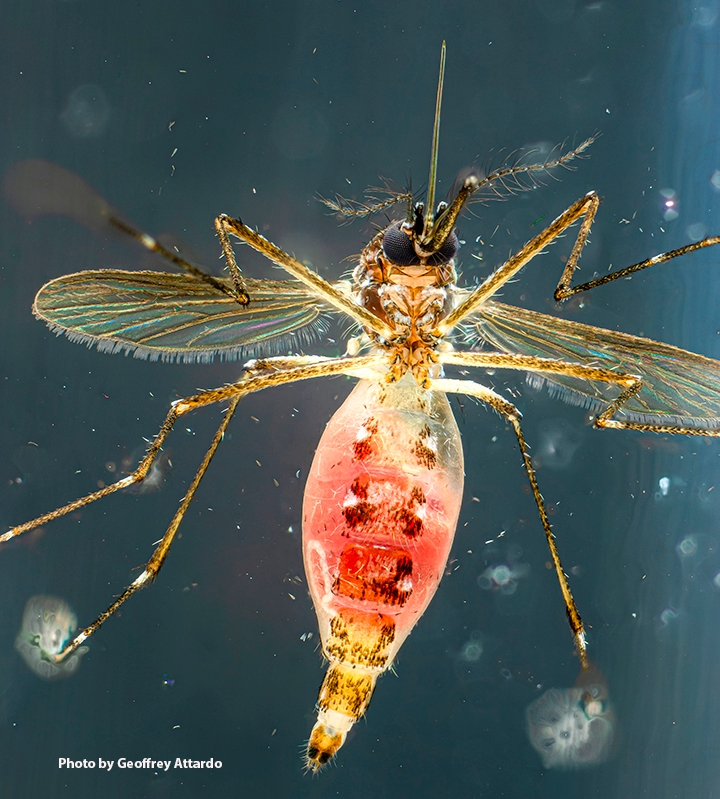This magnified photograph vividly captures the intricate details of a mosquito after it has fed. Its abdomen, now swollen and reddish, indicates that it has recently consumed blood. The body of the mosquito showcases a semi-translucent quality with brown specks scattered within, giving it a somewhat opaque appearance. Its wings are delicate and clear, framed with a brownish hue, and exhibit a subtle goldish tint under the light. The mosquito's six brown legs are clearly visible, as are its two antennae and its needle-like proboscis, which it uses for feeding. The head is predominantly black, and the compound eyes can be discerned, adding to the detailed portrayal of this blood-sucking insect. The photograph is set against an aqua blue, square background, accentuated by specks of white that add a touch of luminosity to the image. The name "Jeffrey Attardo" is noted in white font at the bottom, attributing the remarkable close-up to the photographer.